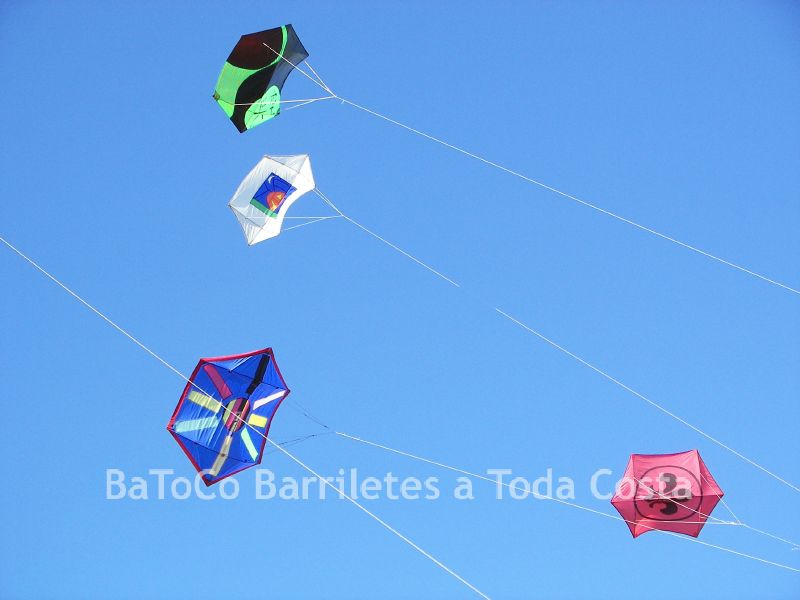A photograph captures a clear, bright blue sky devoid of any clouds or birds, with four colorful hexagon-shaped kites soaring gracefully. At the top center-left, a kite with a fluid pattern of black and light green swirls commands attention, its string reaching across, merging into the others in intricate lines. Just below it, another hexagonal kite stands out with a white background adorned by a blue square and an intricate orange and yellow figure in the center. The third kite, positioned centrally, is striking with its deep blue color, bold red border, and a complex design of multicolored stripes and rectangles converging, resembling a radiant sun. Finally, the fourth kite, located in the lower right-hand corner, is bright red with a distinctive black fleur-de-lis symbol at its core and "BATOC BARILETES A TODA COSTA" written in light blue letters. Each kite is tethered by strings that trace a path through the clear, calm sky, weaving a harmonious pattern in the air. A mysterious fifth string crosses from left to right, its attached kite unseen, adding an element of curiosity to the scene.